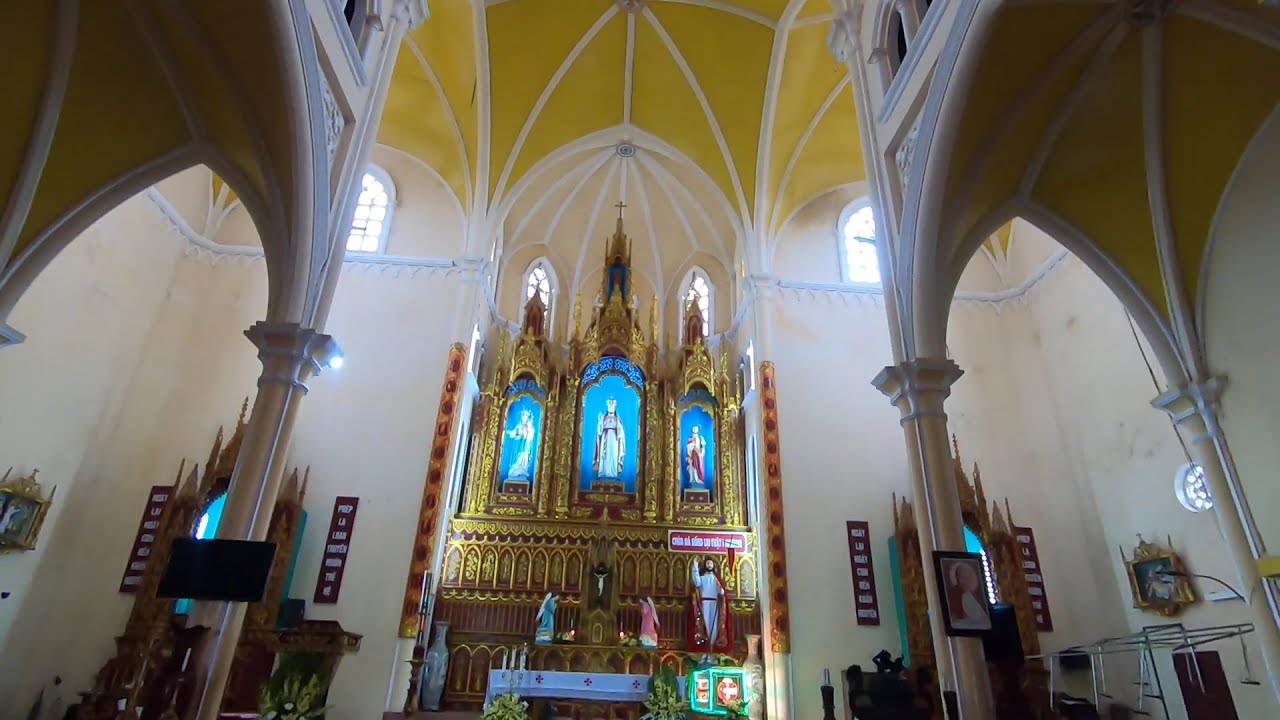This image captures the intricate interior of a church, possibly Catholic or Orthodox Christian. The focus is on the ornate altar and the striking ceiling above it. The church's ceiling is predominantly yellow with white trim, while the walls are a cream or tan color. The altar, a central feature of the image, is opulently gilded in gold with accents of red paint. Centered above the altar is a cross, flanked by two gilded and decorated glass windows indicating it is daytime.

The altar itself is adorned with three prominent statues set against blue backgrounds, likely representing Jesus, the Virgin Mary, and possibly another saint. Beneath this platform, there is a vivid depiction or statue of Jesus on the cross. Surrounding this focal area are additional statues and various religious icons. The detailed artistry extends to various paintings and signboards on the church walls, contributing to the church's rich, sacred ambiance. Notably, the scene is devoid of people, emphasizing the spiritual and solemn atmosphere of this holy place.